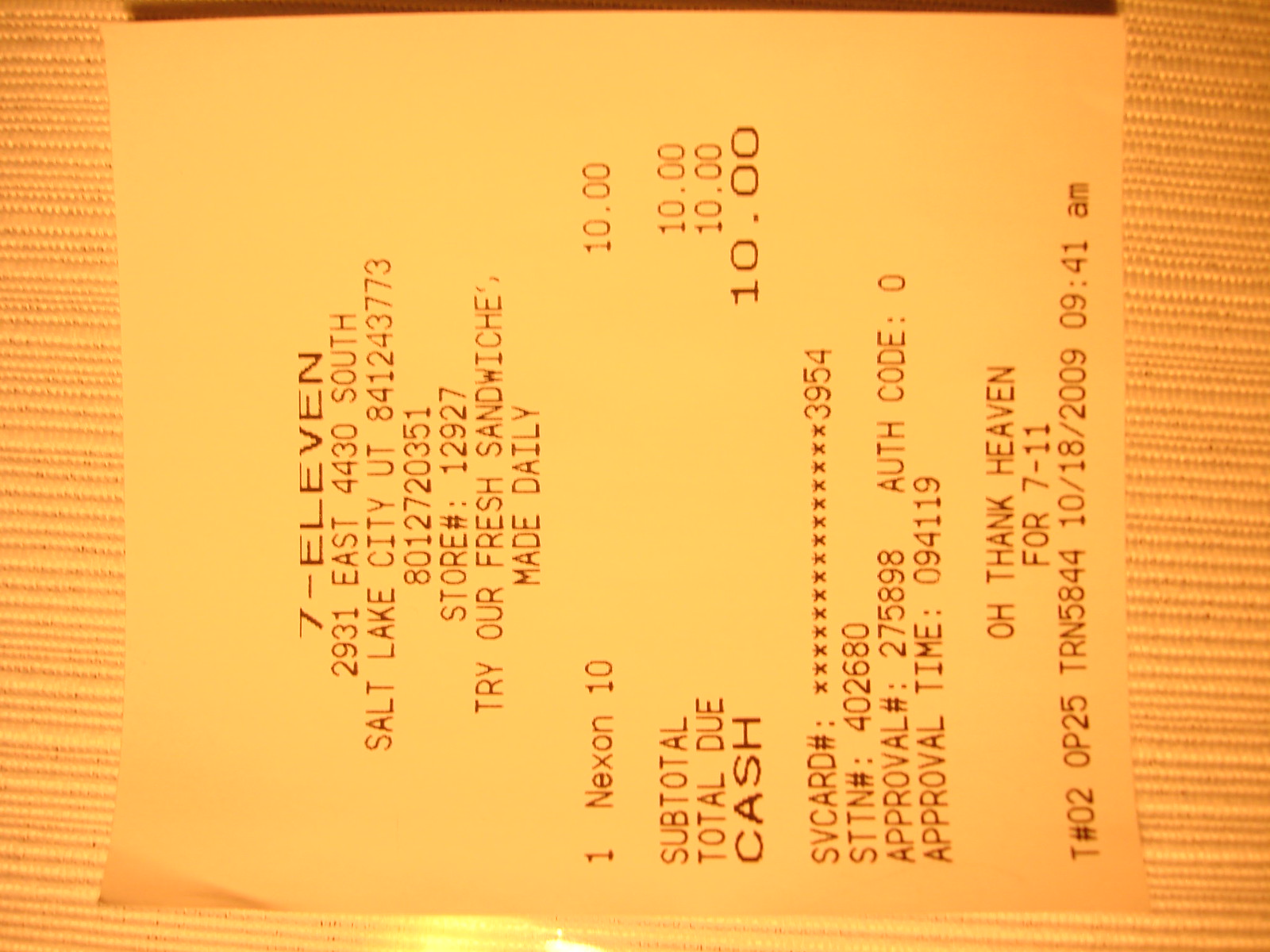The photograph depicts a small, sideways receipt from a 7-Eleven store. The receipt's header displays the store's address: "7-11, 2931 East 4430 South, Salt Lake City, Utah," followed by additional numerical identifiers including the store number. A promotional message prominently encourages customers to "try our fresh sandwiches made daily." Below the promotional message, a purchase of "one Nexon 10" is listed, accompanied by a charge of $10. The financial breakdown details a subtotal of $10, a total due of $10, and a cash payment of $10. Further information is present at the bottom, concluding with the familiar slogan, "Oh, thank heaven for 7-11."